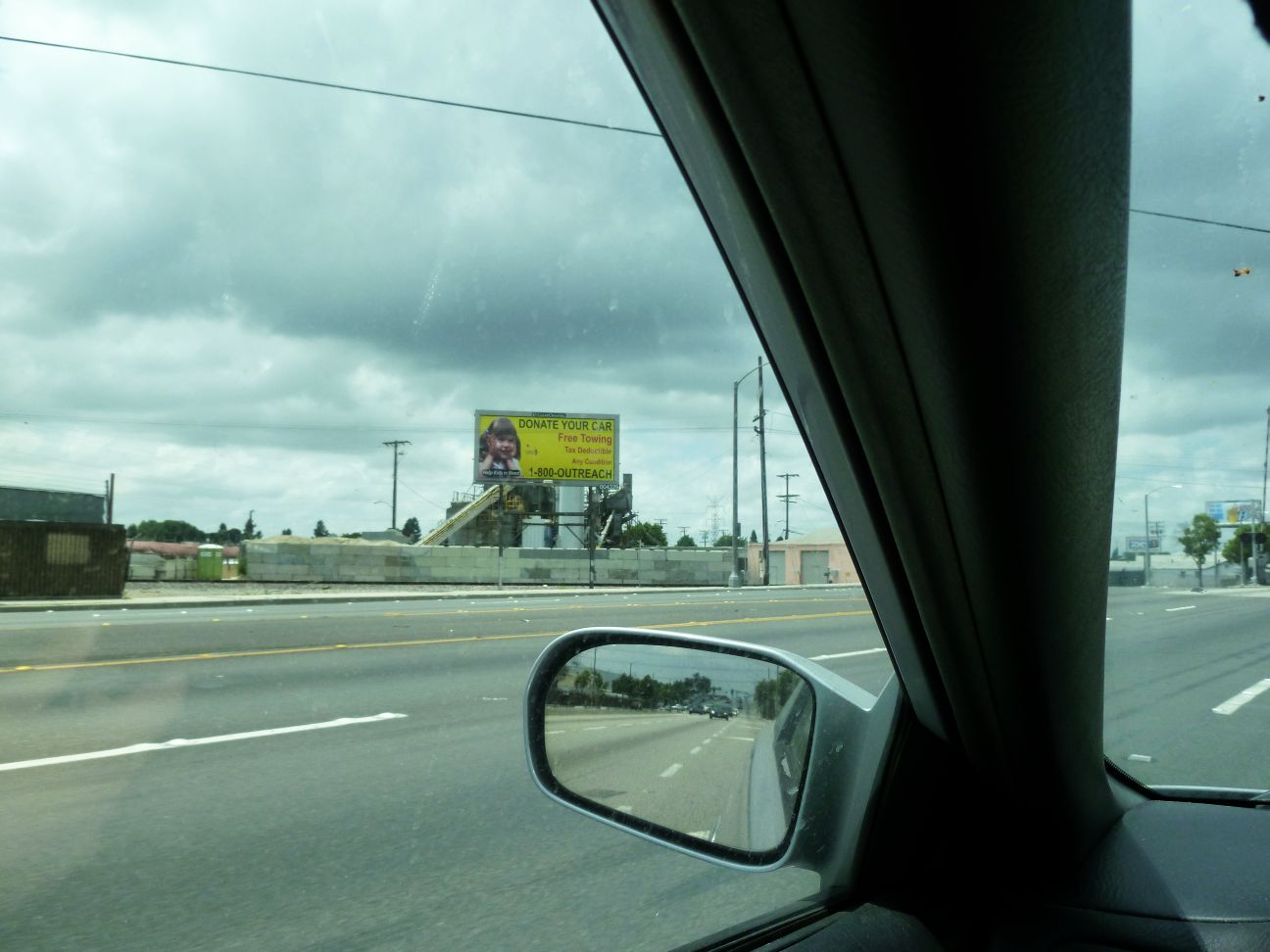This image captures the view from the front corner of a moving car, taken from the driver's seat. The scene unfolds on a wide, six-lane road devoid of other vehicles directly ahead. A solitary car is visible in the rearview mirror. The sky is a blanket of dense, overcast clouds, adding a somber tone to the setting. Dominating the center of the photograph is a yellow billboard that reads, "Donate Your Car, Free Towing," accompanied by an image of a girl's face. Below this billboard stretches a long brick wall. To the right of this wall stands a low-tan building with two garage doors, while to the left lies a smaller, dark building, partially obscuring another structure behind it.